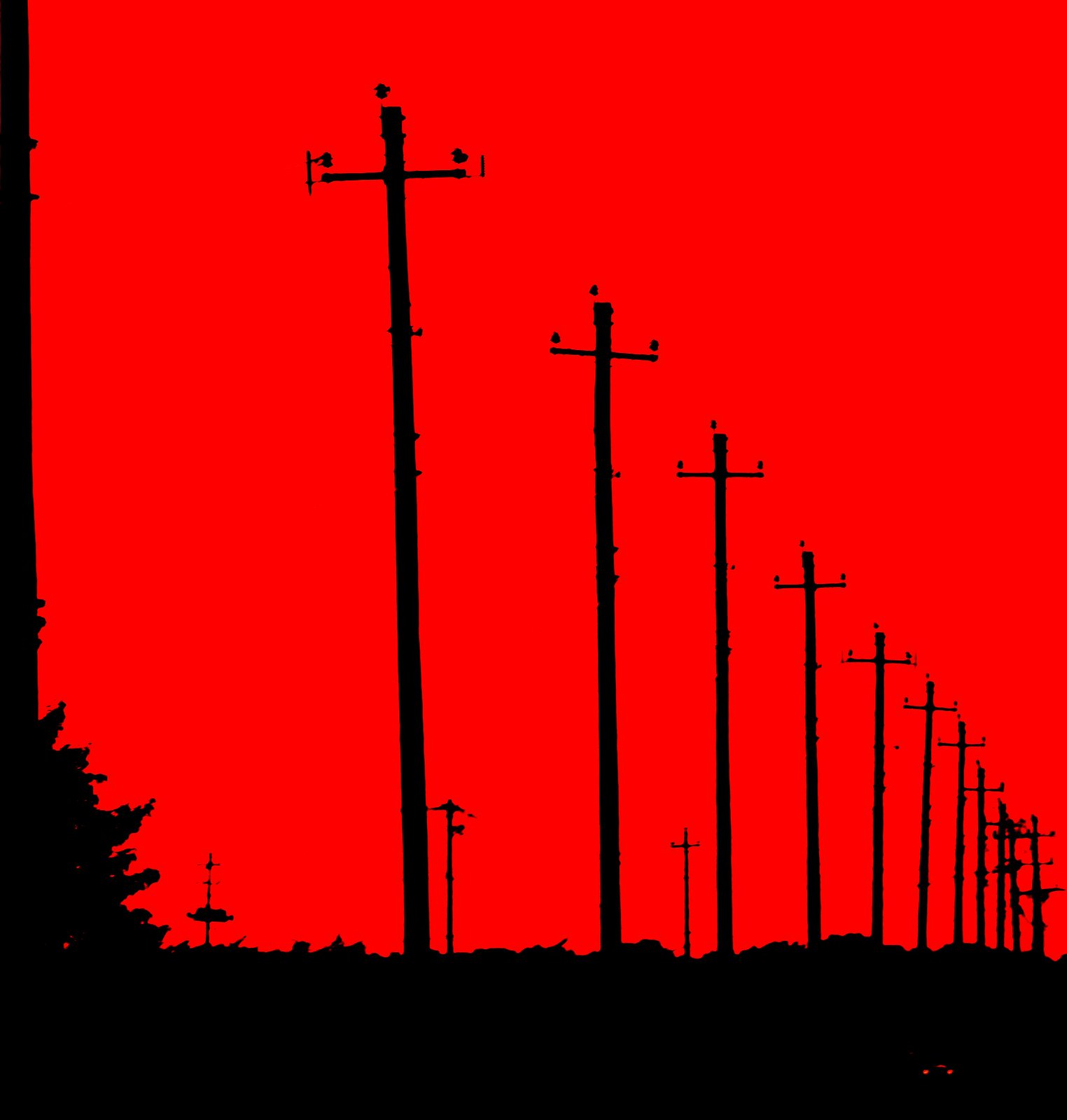This striking vertical image captures a stark and evocative silhouette scene. Dominated by a deep, blood-red background, the foreground is inky black, hinting at a terrain silhouette. The left side features the dark outline of a small bush, or perhaps a distant pine tree. A series of eleven tall utility poles march diagonally from the left to the lower right corner, decreasing in height as they move further away. Each pole supports a horizontal crossbar near the top, extending roughly two feet on either side, reminiscent of runway markers or telephone poles. Insulators and what appear to be lights or small birds dot the tops and crossbars of each pole. The final pole in the distance features three arms, adding a touch of complexity to the scene. The distant background also reveals three additional poles in a separate line, with one possibly cradling a bird's nest. The uniform red background and the striking black silhouettes create a hauntingly beautiful visual.